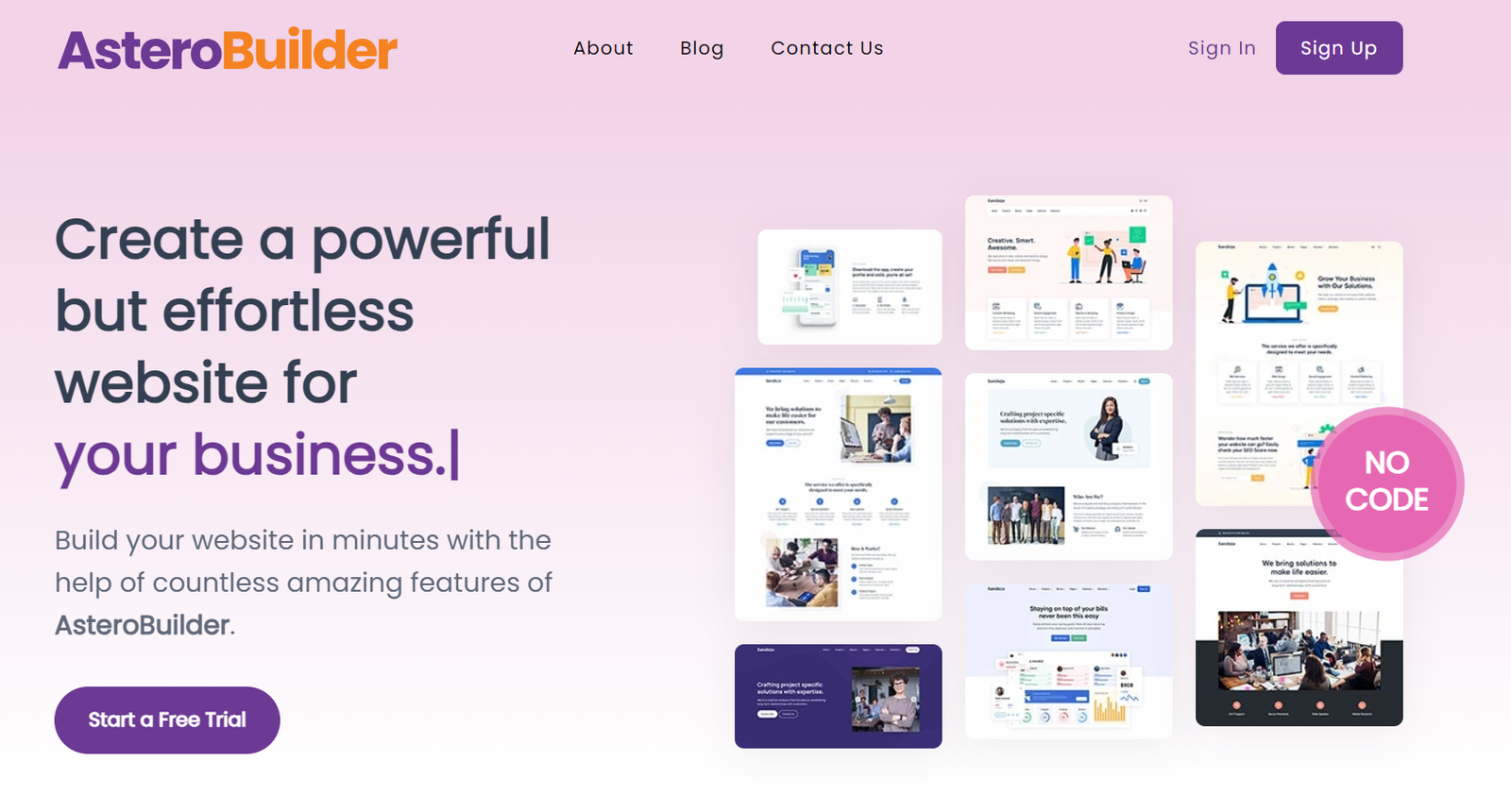AstroBuilder: Effortlessly Create a Powerful Website for Your Business

AstroBuilder invites you to build your website in minutes with its extensive array of amazing features. The "No Code" label is prominently displayed inside a giant pink circle, emphasizing ease of use. On the right side of the image, there are eight screenshots showcasing various websites crafted using AstroBuilder, highlighting its versatility. The "Sign Up" button features a striking design with purple text on a purple square background, making it stand out.

In the top left corner, the word "Astro" is written in a stylish purple font, formatted as A-S-T-E-R-O, paired with "Builder" in a vibrant orange. "Start a Free Trial" is emphasized with a pill-shaped, purple-colored background to catch the viewer’s eye. The bottom half of the background is white, gradually transitioning into a soft pink hue towards the top, adding a subtle yet appealing gradient effect. Additionally, navigation links like "About," "Blog," "Contact Us," "Sign In," and "Sign Up" are available, ensuring accessibility and ease of use for visitors.